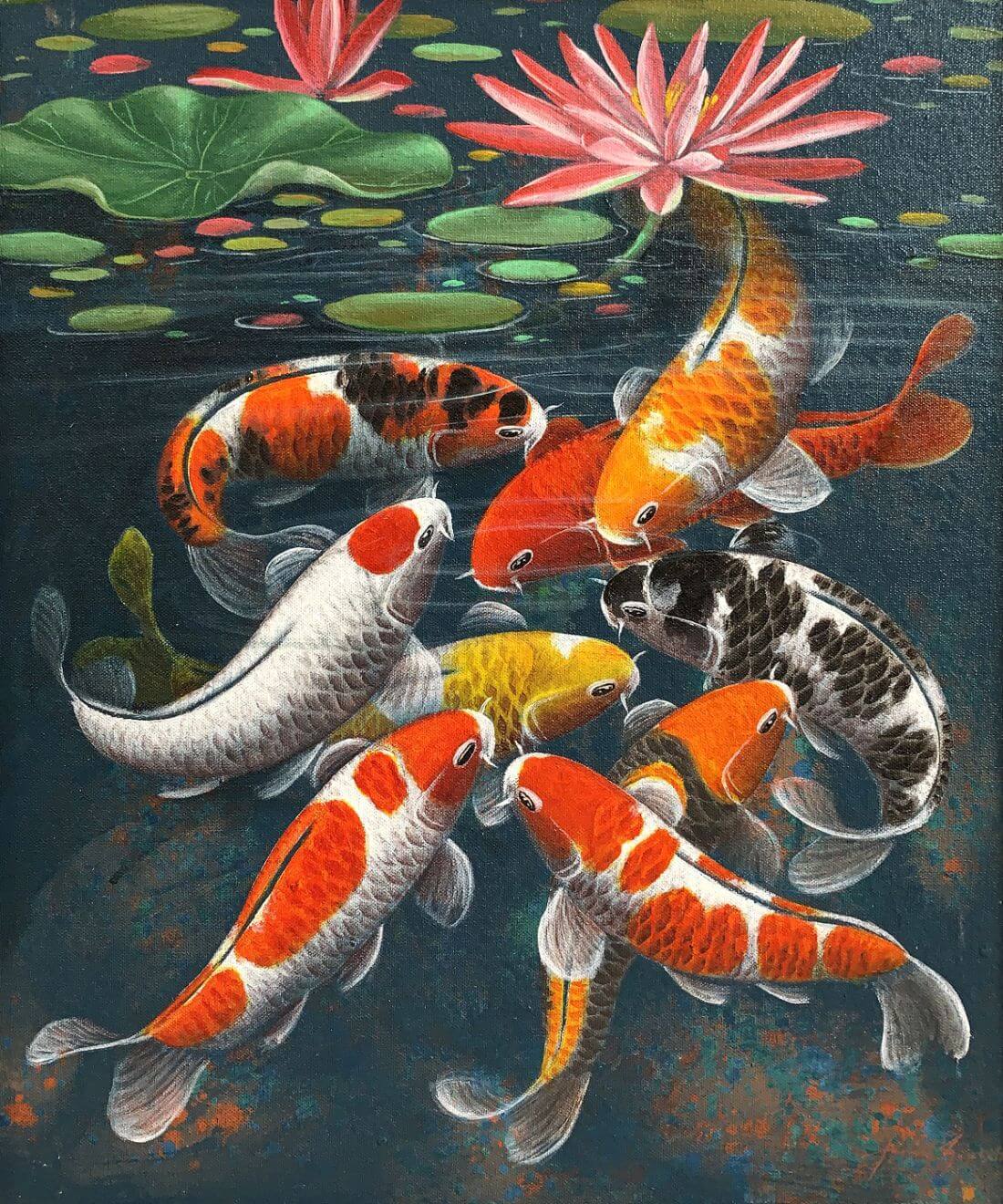This detailed color illustration captures a tranquil koi pond filled with vibrant aquatic life. The water is painted in deep, dark blue hues, its surface subtly suggested by white lines that hint at reflections. Floating serenely on the water are several green lily pads, interspersed with blossoms in shades of pink and yellow, and a couple of striking reddish flowers. Beneath the surface, the composition is teeming with activity as approximately a dozen koi swim in a crowded, swirling dance. Among them, there are two koi with gold and white scales, three in orange and white, and a colorful mix featuring orange, black, and silver hues. Adding to this palette, there’s a black and white koi, another in a blend of orange, black, and white, and a distinctive white koi with a prominent red dot on its head. The illustration captures the koi in varying poses, contributing to a sense of dynamic movement within the serene environment.